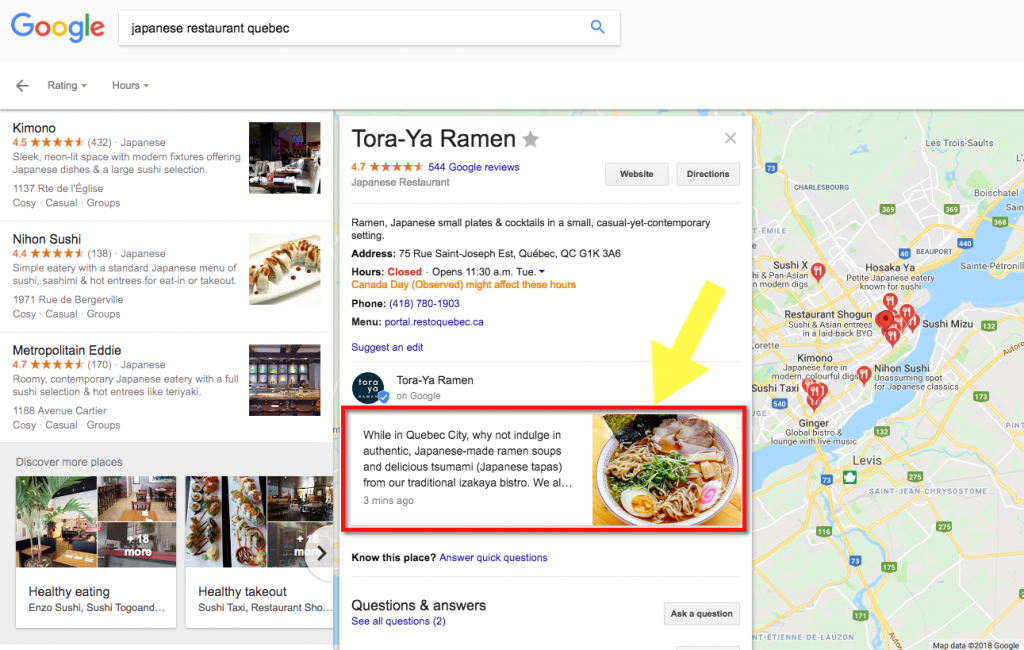This image captures the screen of a Google search result for "Japanese Restaurant Quebec." The image is in portrait orientation, with no defined borders. 

At the top, there is a horizontal gray bar featuring the Google logo in the upper left corner, adjacent to a long, rectangular white search box that contains the black text “Japanese Restaurant Quebec.” Directly below, a white bar includes a back arrow on the left, alongside drop-down menus for ratings and hours to help sort the results.

The search results are displayed in three main sections. On the left, a column showcases various Japanese restaurants with a white background. Each restaurant listing includes a thumbnail image, the establishment name, and its star rating. The results include:
1. Kimono – 4.5 stars
2. Neon Sushi – 4.4 stars
3. Metropolitan Eddie – 4.7 stars

At the bottom of this column, there is a gray box offering additional options like "Discover More Places," "Healthy Eating," and "Healthy Takeout."

The middle section prominently features a detailed result for Toriya Ramen, rated 4.7 stars. This segment provides essential information such as the restaurant’s address, hours, phone number, menu, and a link to Google reviews. It includes an image of ramen enclosed in a red rectangular box with a border, accompanied by a yellow arrow pointing downward, likely to draw attention to this specific result.

On the right side of the screen, there is a map marking the locations of all the listed restaurants, giving users a visual representation of their options.

This detailed layout helps users to easily browse through options, compare ratings, and gather necessary information to make an informed decision about Japanese dining in Quebec.